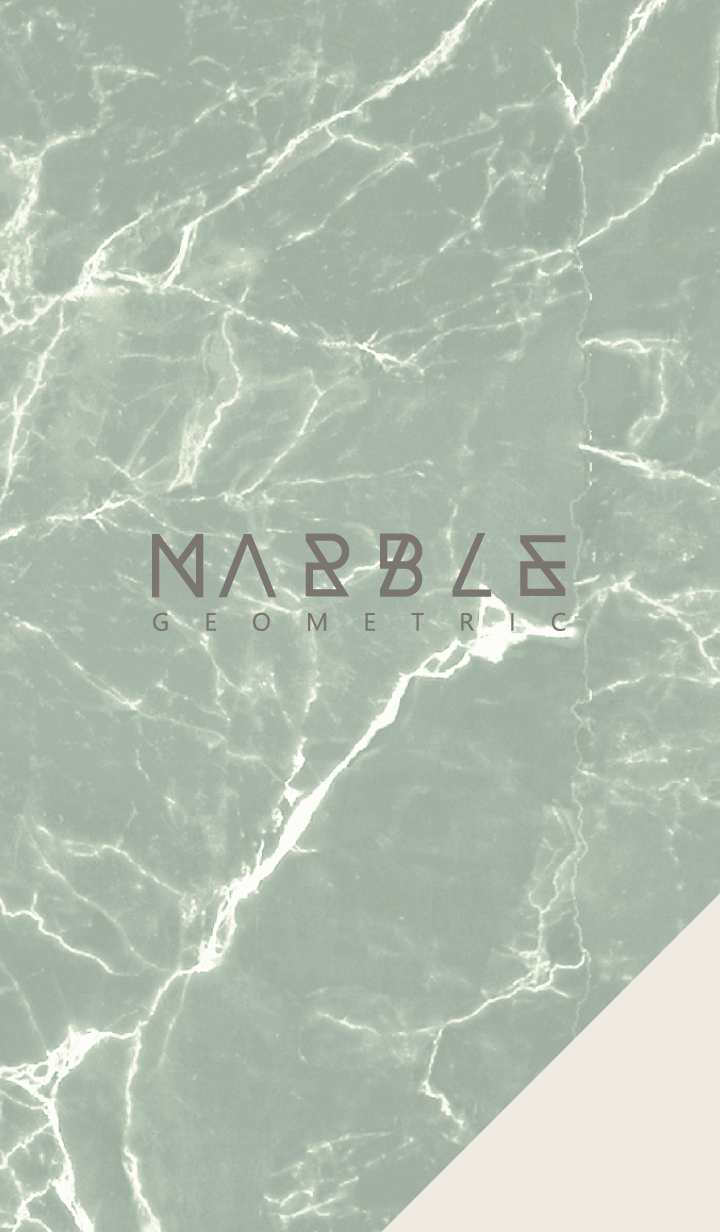The image features what appears to be a front cover of a book, magazine, or potentially a music album, showcasing a minimalist and modern design. The background is a light mossy green marble with intricate white veining that mimics the refracted sunlight on a clear body of water, giving it a serene, aquatic feel. Centered in the image is a logo with the word "MARBLE" in a dark gray, architectural-looking font. Below it, in a slightly different font, the word "GEOMETRIC" is displayed in the same color. The marble background extends throughout the top section of the image, with a distinct light gray triangle cut out of the bottom right corner, which is pure white, separated by a diagonal line. The overall aesthetic of the image blends elements of nature with sleek, geometric typography, suggesting a sophisticated, upscale design, akin to the countertop of a modern kitchen or an elegant piece of green marble.